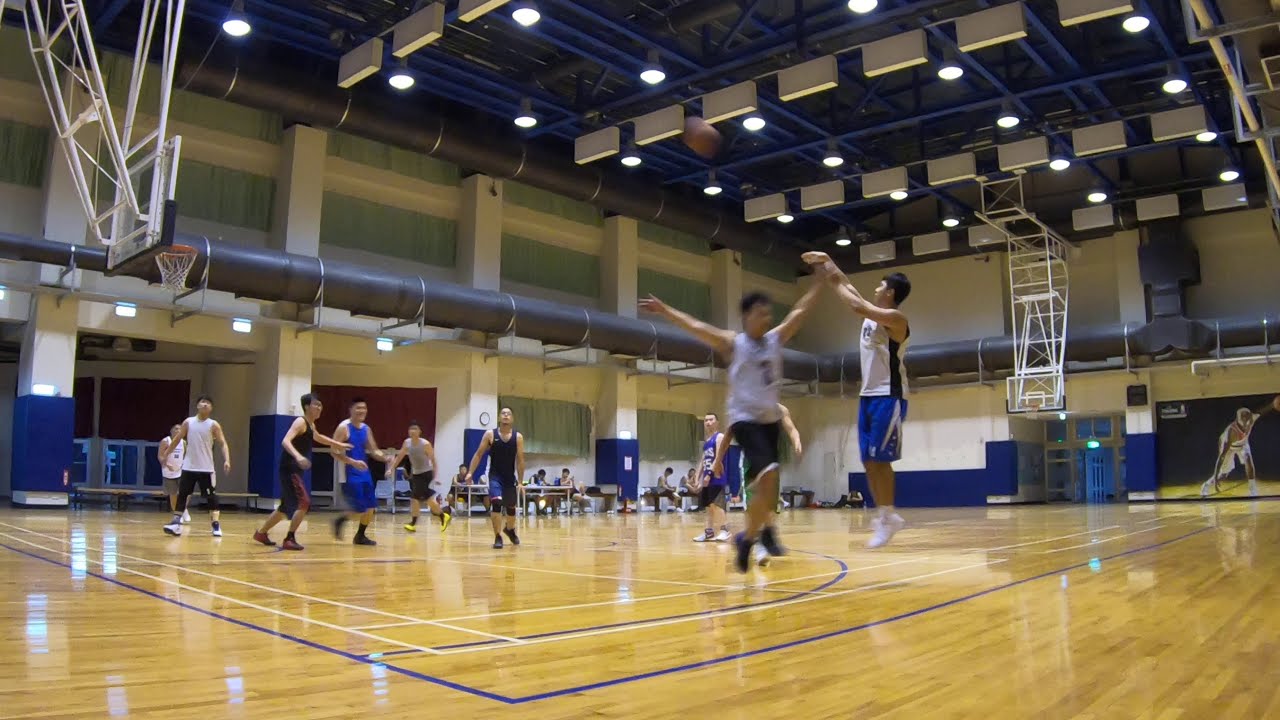The image depicts a lively recreational basketball game taking place in what appears to be a high school gymnasium. To the center right, a player in a white jersey and blue shorts is captured mid-jump with his right arm extended, releasing the ball into the air for a three-point attempt. To his left, an opponent in a gray shirt and black shorts leaps in an unsuccessful attempt to block the shot. Behind the jumping player in gray, another participant’s left arm is visible, partially obscured by the action. Further to the left, another player in a blue shirt looks on. The court is bustling with six additional players, wearing a mix of black, gray, blue, and white shirts. Amidst the action, the gym’s wooden floor is marked with white and blue taped lines. In the background, a group of individuals, possibly spectators or scorekeepers, sit against the wall beside a table, observing the game unfold. The lack of official uniforms and the casual attire suggest this is a recreational league tournament, focused more on the spirit of play than formal competition.